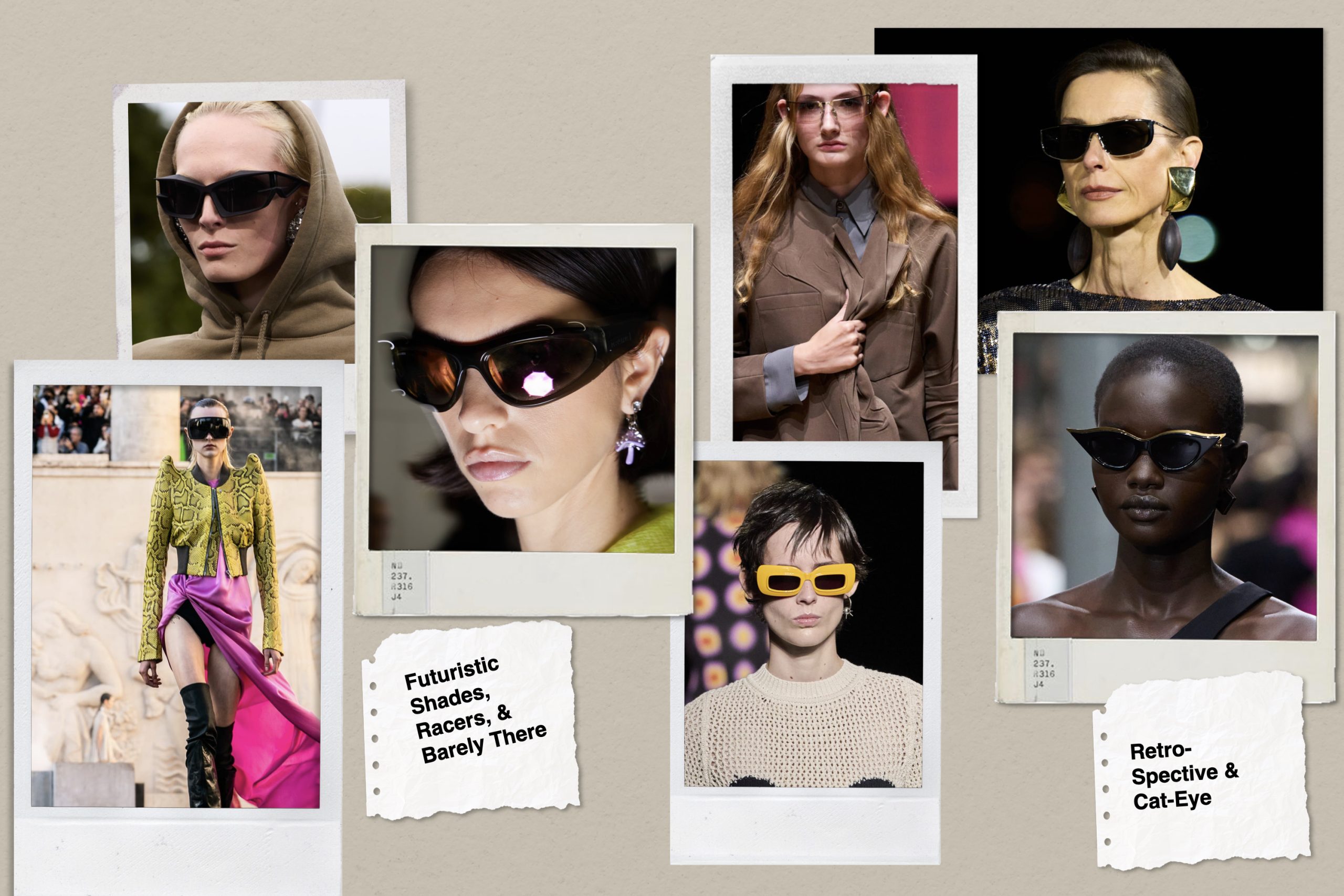This image is a computerized collage of real photos of women showcasing various styles of sunglasses, positioned as if pinned to a bulletin board. The display mimics Polaroid photos with a vintage yet modern aesthetic. At the top left, a woman with blonde hair wears glasses and a dark tan hoodie. Below her, a woman strides forward in a yellow shirt with oversized puffy shoulder pads, a purple skirt, and thigh-high black boots, sporting large glasses or a mask. To the right, another woman in glasses faces left, above a slip of paper reading "Futuristic Shades, Racers and Barely There." In the top center, a woman in a brown coat wears regular glasses, while beneath her, a woman with short black hair dons yellow-tinted glasses. At the top right, an older woman with large earrings faces left, wearing glasses. Beneath her, another woman displays cat-eye glasses with a flare at the top. At the very bottom right, a note reads "Retrospective and Cat Eye." The sunglasses range widely in style, color, and frame thickness, from thick-rimmed to barely-there, embracing both futuristic and retro themes on a brown background.